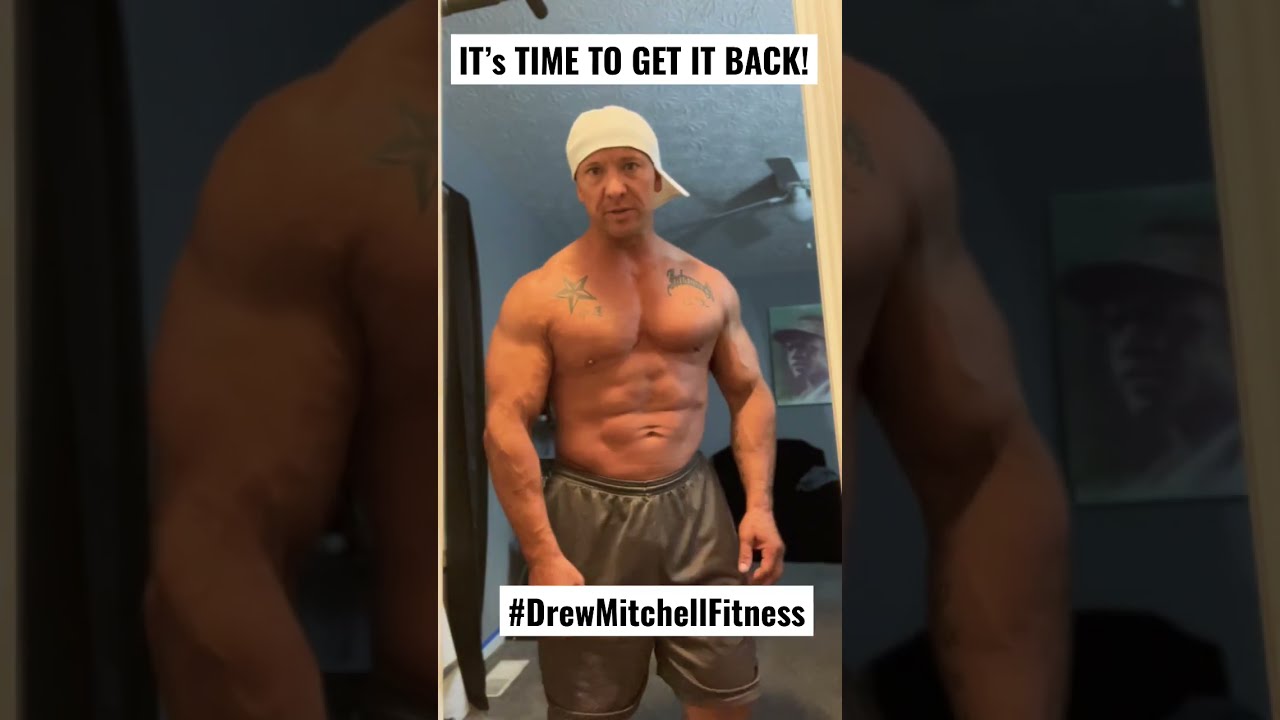This is a detailed color photograph of a shirtless, muscular middle-aged man who appears to be a bodybuilder, showcasing his well-defined physique and six-pack abs. He has tattoos on his chest and shoulders, including a star and some indecipherable text. He is wearing a white baseball cap turned backwards and loose, grayish shorts. He stands confidently in front of a white wall, next to a black bag and some small boxed items, likely in the doorway of a bedroom with a ceiling fan visible and gray walls in the living room area. The image has a portiform orientation and is inset into a background photograph of the same image, but darkened and in landscape orientation. The top of the image reads "It's time to get it back!" in bold, all-caps black text on a white strip, while the bottom reads "#Drew Mitchell Fitness" in bold black text with mixed capitalization. The overall style of the photograph is representational realism.